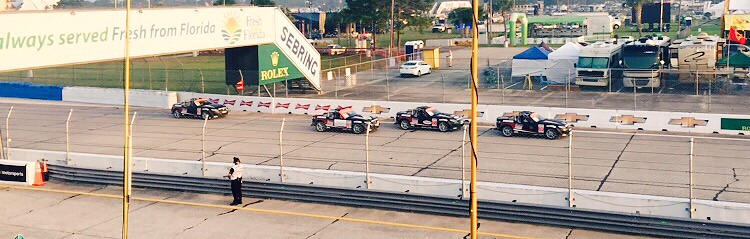The photograph, taken on a sunny day outdoors, captures a wide, horizontally rectangular view of a racetrack with a light gray paved surface that starts slightly in the middle of the left side and tilts down towards the bottom right, appearing wider as it extends to the right. The track is bordered by white barriers on either side. Above the track, visible signage includes a banner reading “Always served fresh from Florida” accompanied by the Fresh Florida logo, the word "Sebring," and a green Rolex sign. 

Four black sports cars, heavily adorned with logos and possibly Corvettes or convertibles, are staged to start a race, lined up against the small white wall with Chevrolet and Budweiser branding. Nearby, a race official in a reflective safety vest stands behind the barrier, watching the cars. Two large yellow poles, partially visible, are located in the foreground of the image.

In the background, beyond the track, a parking lot filled with various vehicles, including RVs and tents, is visible. Further in the distance, a green and white stage suggests a carnival-like event with board parties and concession stands, adding to the lively atmosphere. Despite the detailed setting, there is no visible audience in the scene. The image conveys the excitement and preparation at the start of a significant race event.